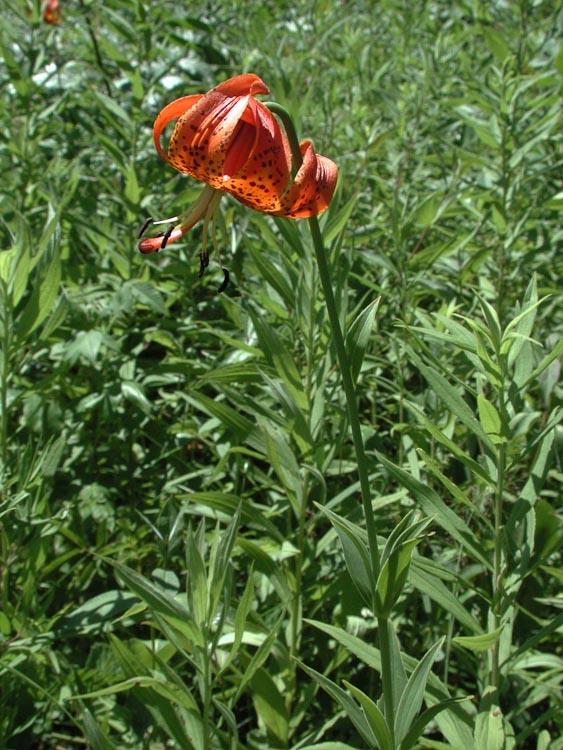This photograph, in a portrait layout, captures a lush, vibrant field teeming with greenery, grass, and various wild plants. Dominating the center of the image is a striking, orangey-red flower connected to a long, slender green stem that extends downward to the lower right corner. The flower, characterized by different shades of red, orange, and coral, features darker spots and tiny seed pods. Enhancing the serene ambiance, another blurred red flower is subtly visible in the far upper left corner. The surrounding vegetation consists of a variety of green weeds, grass, and additional flowers, possibly including tiger lilies. The image exudes the feeling of a sunny day, as the flower glistens softly in the light. The scene lacks any human presence, focusing instead entirely on the natural beauty of this wild field.